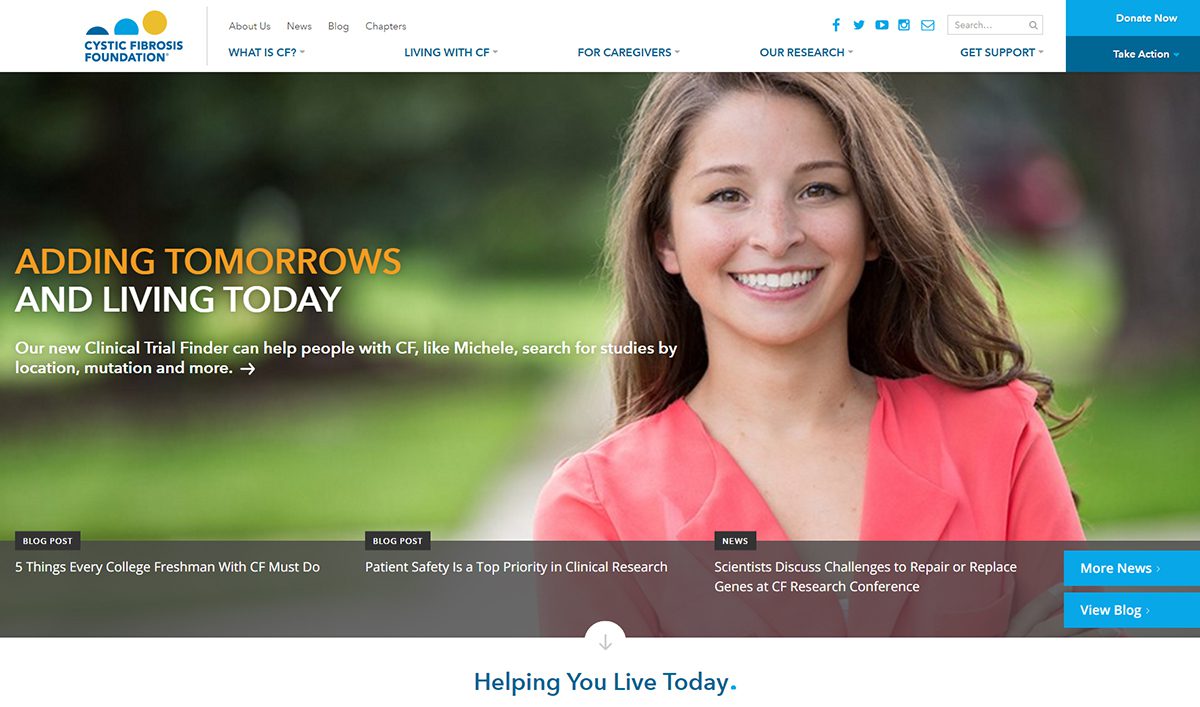The main page of the Cystic Fibrosis Foundation website prominently features a young woman named Michelle, who is smiling brightly. Michelle, who has brown hair and is wearing a chic pink suit top with a barely visible undershirt, exudes happiness and high spirits. She is standing on a cement path surrounded by trees and grass, suggesting the photo was taken in a park. Michelle's beaming smile showcases her beautiful teeth, adding to her radiant appearance.

To the left of Michelle's image, the text "Adding Tomorrows" is displayed, emphasizing the foundation's mission. The page header includes the Cystic Fibrosis Foundation logo, represented by several ball icons. Navigation links at the top of the page offer sections titled 'What is CF,' 'Living with CF,' 'Caregivers,' 'Research,' and 'Get Support.' Additionally, there is a search bar, social media links, and an 'About Us,' 'News,' 'Blog,' and 'Chapters' sections.

Alongside Michelle's photo, a message reads, "Adding Tomorrow and Living Today. Our new clinical trial finder can help people with CF like Michelle search for studies by location, mutation, and more." This indicates that Michelle is likely a person living with CF and is featured to highlight the foundation's clinical trial finder tool.

At the bottom of the page, further sections include blog posts such as "Five Things Every College Freshman with CF Must Do," "Patient Safety is Top Priority in Clinical Research," and "Scientists Discuss Challenges to Repair or Replace Genes at CF Research Conference," providing valuable information and updates to the CF community.